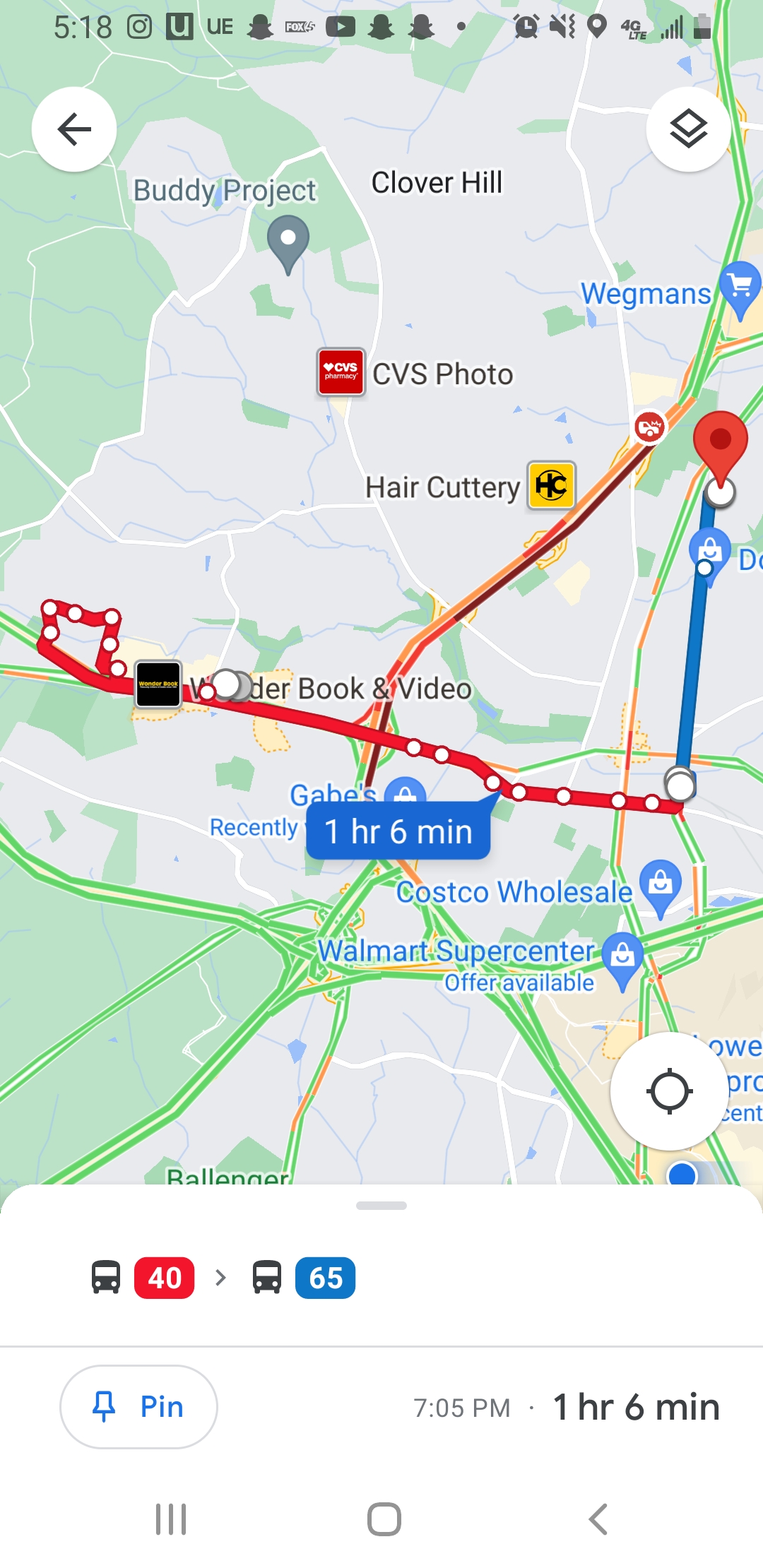The image is a screenshot from a maps application, likely Google Maps, on a mobile device or car navigation system. The map displays a mix of green and gray areas representing a cityscape and natural terrain. Red and blue lines trace the route, forming an L-shape that heads south before turning west. This route is marked by a blue arrow and box indicating it will take 1 hour and 6 minutes to complete. The map also features various roadways in green and orange, and notable locations such as Buddy Project, Clover Hill, CVS Photo, and Haircuttery. At the end of the red route, it continues in blue with a pin marking the destination. The screen shows additional locations like Costco Wholesale and Walmart Supercenter, as well as several map icons and various interface elements indicating the time, notifications, battery status, and a presumed zoom function. There are also bus icons labeled 40 and 65, though their significance is unclear.